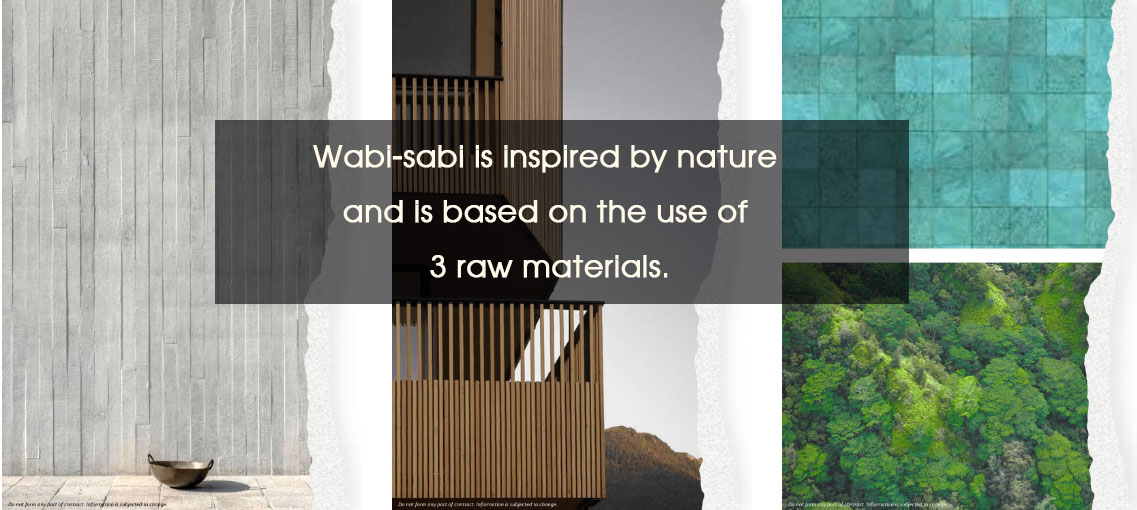The image is a composite of four different photographs arranged side by side, with a translucent gray square in the center that displays white text stating, "Wabi-sabi is inspired by nature and is based on the use of three raw materials." The first photograph on the left features a textured gray wall behind a floor made of a different material, on which a dark brown metal bowl with two handles is placed. The second photograph captures the corner of an exterior house structure showcasing bamboo-like sticks used for the walls and a balcony. The third photograph, in a split layout, shows two smaller images stacked vertically: the top half depicts a surface in a turquoise color, which could be a wall or floor, while the bottom half presents an aerial view of lush green treetops.